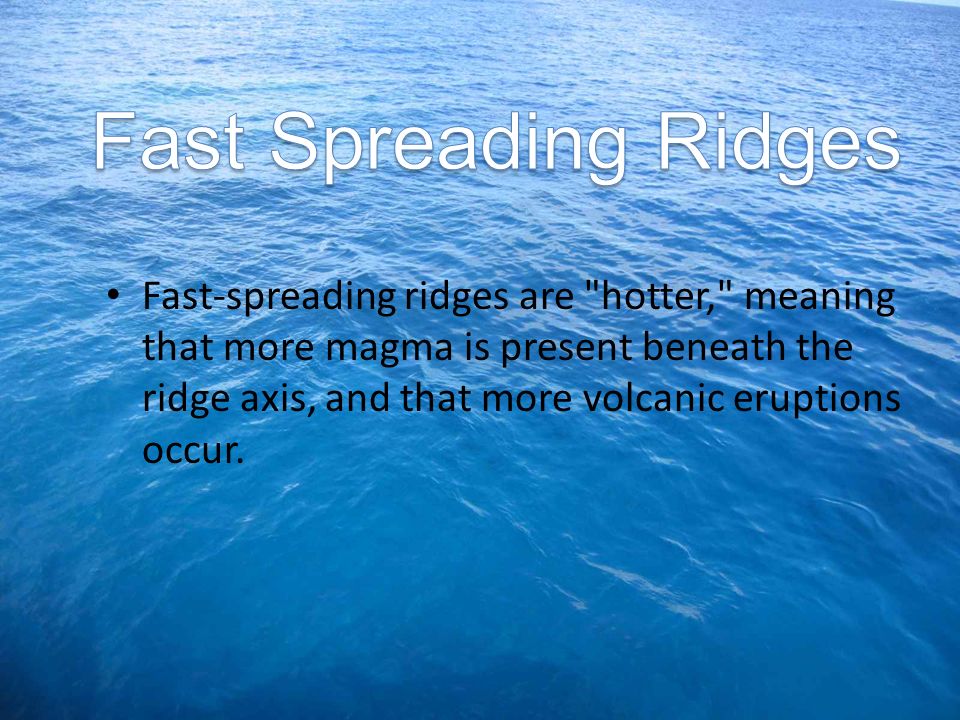The image appears to be a photograph of a PowerPoint slide with the background featuring a vast, rippling body of clear, blue ocean water under a sunny sky. The water is darker blue at the bottom and gradually shifts to a lighter blue towards the top. The title "Fast Spreading Ridges" is prominently displayed in white text at the top of the slide, with a bold black outline to enhance its visibility. Below the title, a bullet point in black text reads, "Fast Spreading Ridges are hotter, meaning that more magma is present beneath the ridge axis and that more volcanic eruptions occur." This text overlaid on the serene ocean image emphasizes the geological concept being discussed, suggesting that volcanic activity can take place beneath these underwater ridges.